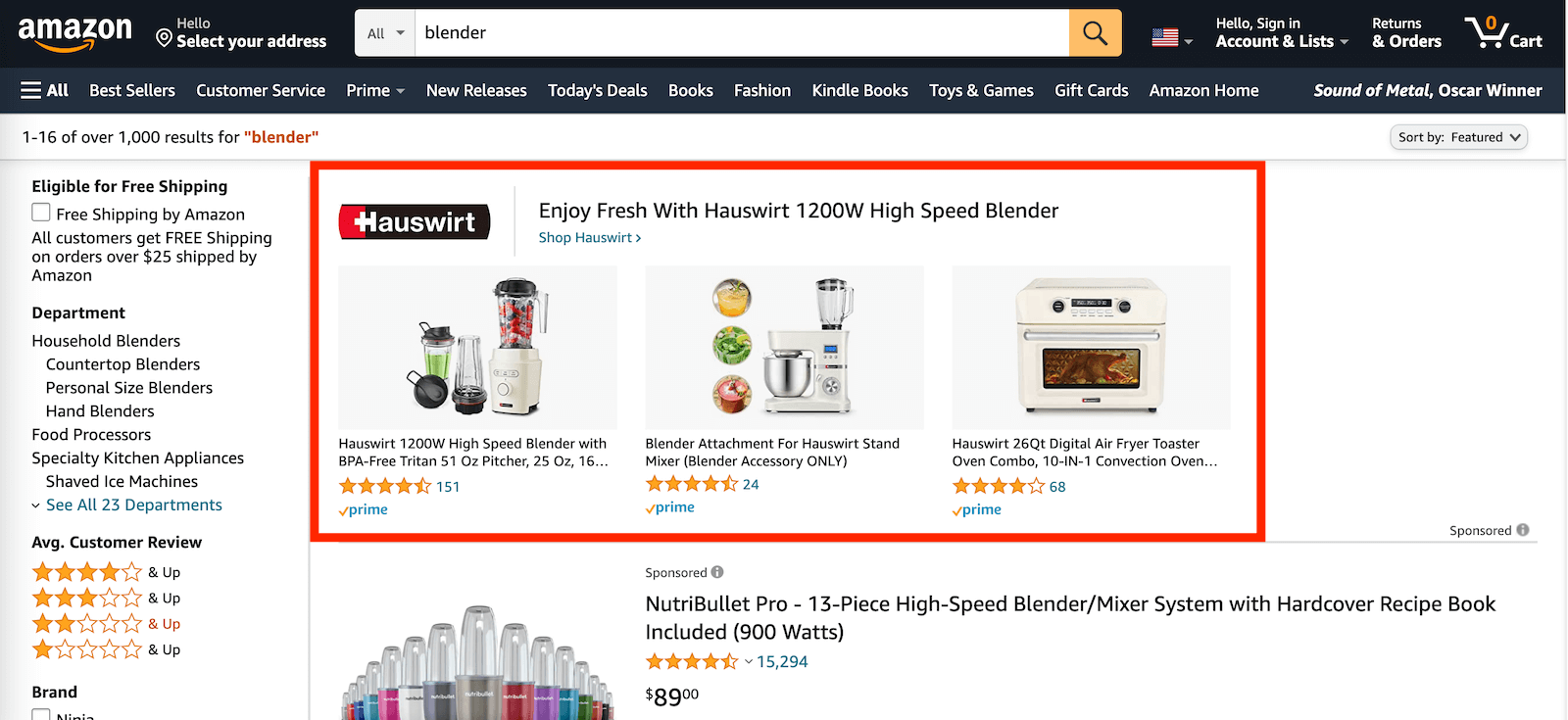A screenshot captured from a desktop or iPad, judging by the dimensions, depicting the Amazon main page. While the URL is not visible, the Amazon logo is clearly positioned on the top left, adjacent to the prompt "Hello, select your address." Below the logo is the search bar set to "All" as the drop-down category menu, with the user having searched for "Blender." The top right shows options "Hello, sign in," "Account & Lists," "Returns & Orders," and "Cart," indicating no user is signed in. The displayed search results feature various blenders, with the first result highlighted by a red border. This primary result showcases the brand "Housewood," with the title "Enjoy Fresh with Housewood 1200 Watt High-Speed Blender." Accompanying the title are images of two different blenders and one item resembling an air fryer toaster, each with corresponding descriptions beneath them.